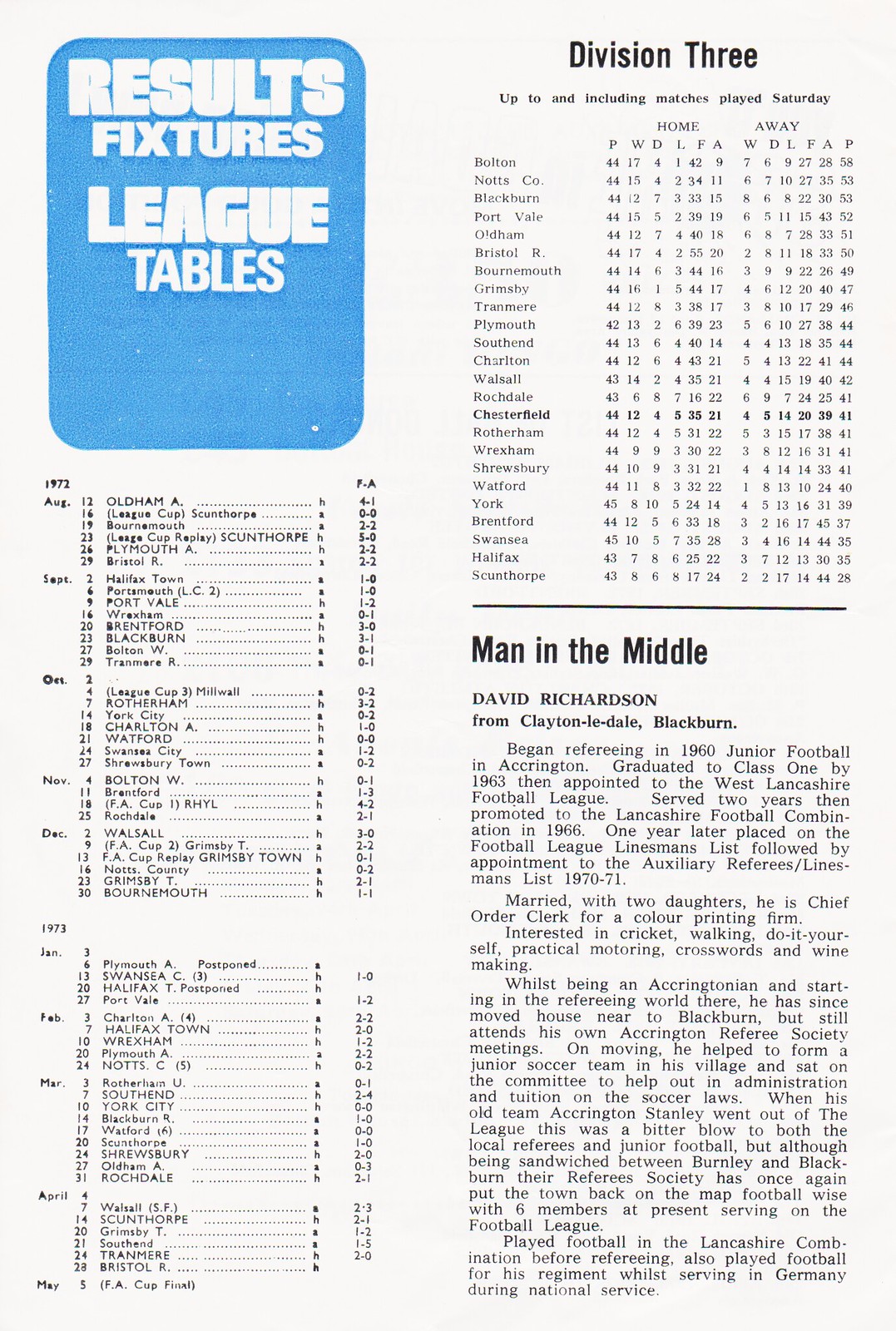This image is a detailed rectangular league results table and summary taken from a sports program or magazine. The design predominantly features a white background with black print, much like a traditional newspaper. In the top left corner, there's a prominent light blue rectangle with white text that reads "Results, Fixtures, League Tables." Adjacent to this, on the right side of the rectangle, is a section titled "Division Three," containing listings of different teams along with their home and away statistics, although the details are very small and hard to discern.

Beneath the blue rectangle on the bottom left, there's an index of various game scores or listings spanning several months, starting from August and continuing through December. These listings are for the years 1972 and 1973, though the exact details are difficult to read due to the small font.

In the bottom right of the image, there's a summary section titled "Man in the Middle" by David Richardson from Clayton Liddell Blackburn. This section describes David Richardson's career, noting that he began refereeing junior football in Accrington in 1960, progressed through various leagues, and was placed on the Football League Linesman list by 1966. Additionally, it mentions his personal life, including his marriage and two daughters, his career as a chief order clerk for a color printing firm, and his interests in cricket, walking, do-it-yourself projects, practical motoring, crosswords, and winemaking.